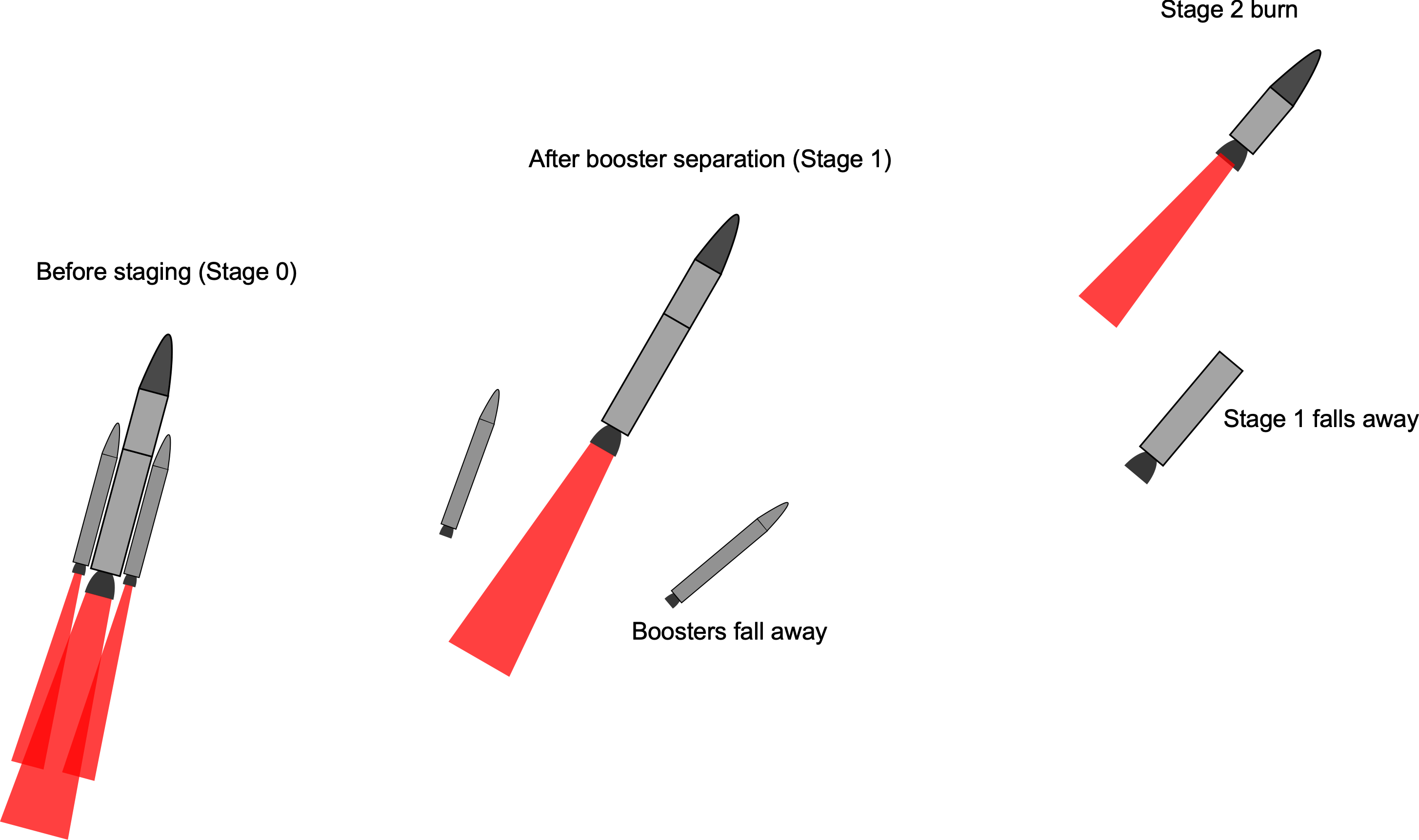The image is a detailed diagram depicting the stages of a rocket launch, set against a plain white background with no visible borders. In the lower left-hand corner, the first stage labeled "Before Staging (Stage 0)" shows a gray cylindrical rocket with a domed nose and two smaller booster rockets attached to its sides, all three emitting red flames. Positioned slightly upward and to the right, the next stage is labeled "After Booster Separation (Stage 1)" and shows the two smaller booster rockets broken away and falling to the ground, while only the central taller rocket continues to fire. This stage also has a subtitle, "Boosters Fall Away." In the final illustration in the upper right-hand corner, labeled "Stage 2 Burn," the diagram shows the bottom half of the central rocket detached and falling away, leaving a smaller rocket with a long flame trail behind it. The subtitle here is "Stage 1 Falls Away," indicating the ongoing ascent of the remaining rocket module.